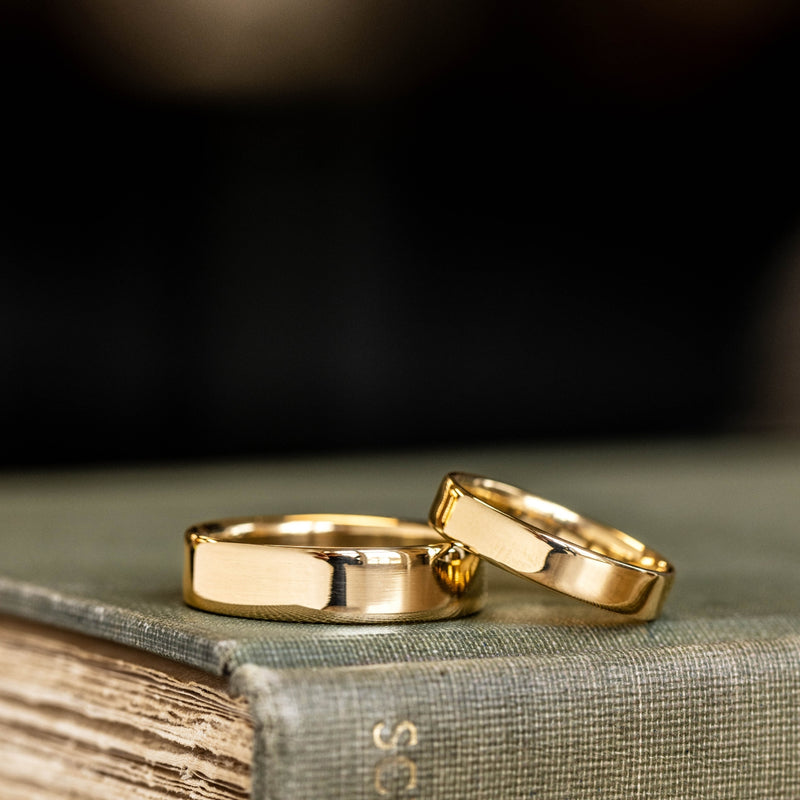This vertical rectangular image depicts the bottom portion of what appears to be a wedding album. The album cover is made of a textured, gray and light tan striped fabric, reminiscent of burlap or tweed. The spine of the album, positioned towards the lower right-hand corner, prominently displays the gold letters "SC." Slightly angled to the right, the album reveals the tops of its frayed pages in the lower left-hand corner, giving it an aged, well-loved appearance.

Resting on the album cover, near the middle of the image, are two gold wedding bands. The larger band lies flat while the smaller band leans on top of it, creating a layered effect. The rings' polished surfaces reflect some light, hinting at the surrounding environment. Above the album cover, the background is completely black, providing a stark but elegant contrast that emphasizes the album and rings.